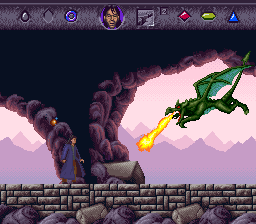A screenshot from a video game depicting an intense moment of action. At the very bottom of the screen lie large, gray rocks forming a rugged terrain. Above this, a rock wall made of similarly gray stones serves as the foundation upon which a character stands. This character, sporting a blue long coat and dark hair, faces right, where a formidable green dragon hovers menacingly. The dragon spews yellow and red fire from its mouth towards the character. The backdrop is a striking contrast: a dark, purplish wall with rocky edges, giving way to distant light purple mountains and a pinkish sky. At the top of the image, game symbols are displayed, including a character’s face and three gems colored red, green, and blue, indicating various game elements.